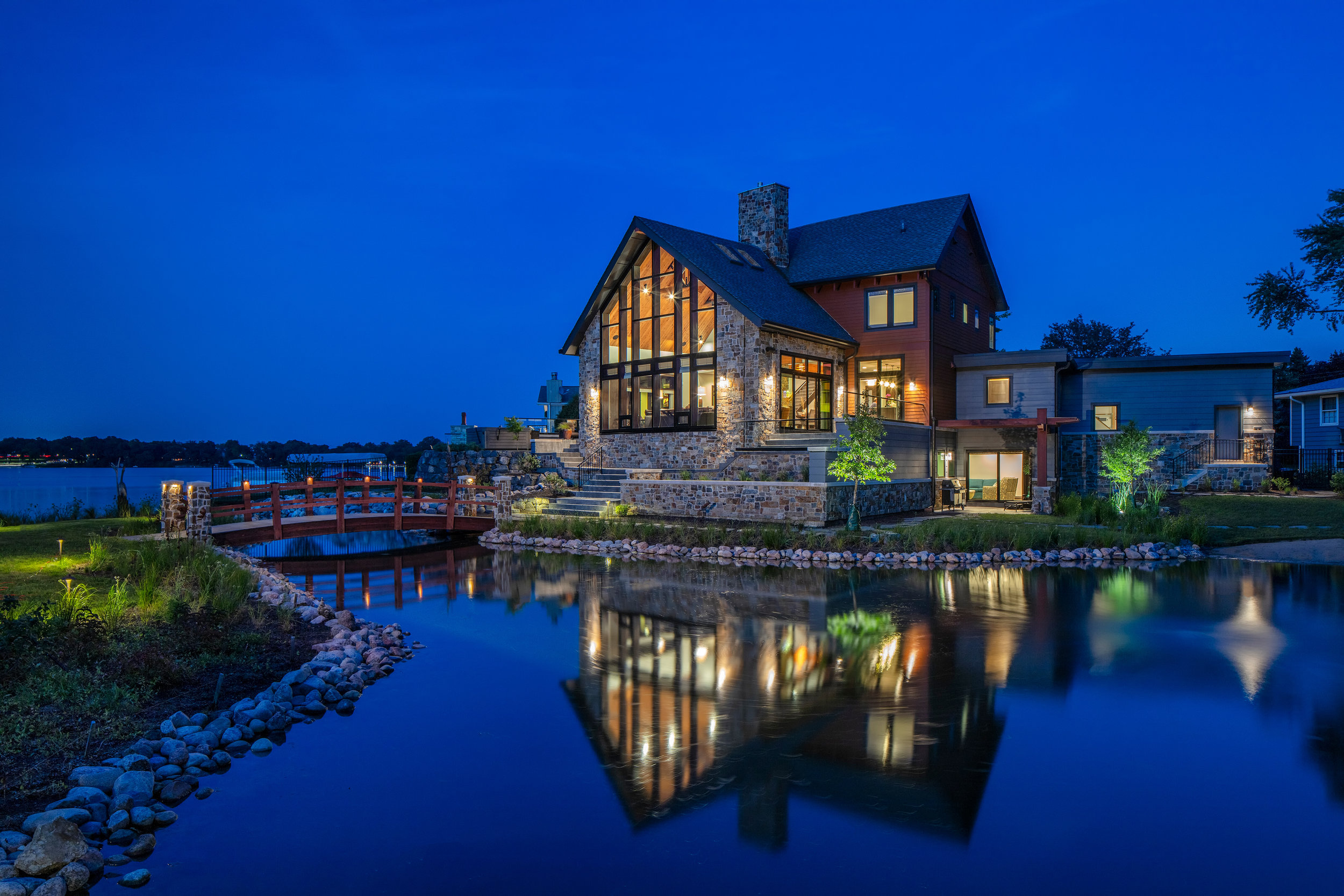A stunning twilight image showcases a modern home with expansive windows, accentuated by electric blue skies. The home features a blend of stone and red siding, with the front predominantly made of glass, showcasing a well-lit interior. A small pond in the foreground reflects the attractive design of the house, while rocks artfully line the water's edge. Surrounding the property, there are trees and a grassy area, and a larger lake can be seen in the distance. The house includes a black roof with skylights and an outdoor area, possibly a garage extension. Notably, a red bridge connects the property to the surrounding landscape. This large, stone-accented home, seen from the backside, reveals intricate details and smaller, unconnected buildings nearby, contributing to the overall picturesque scene.